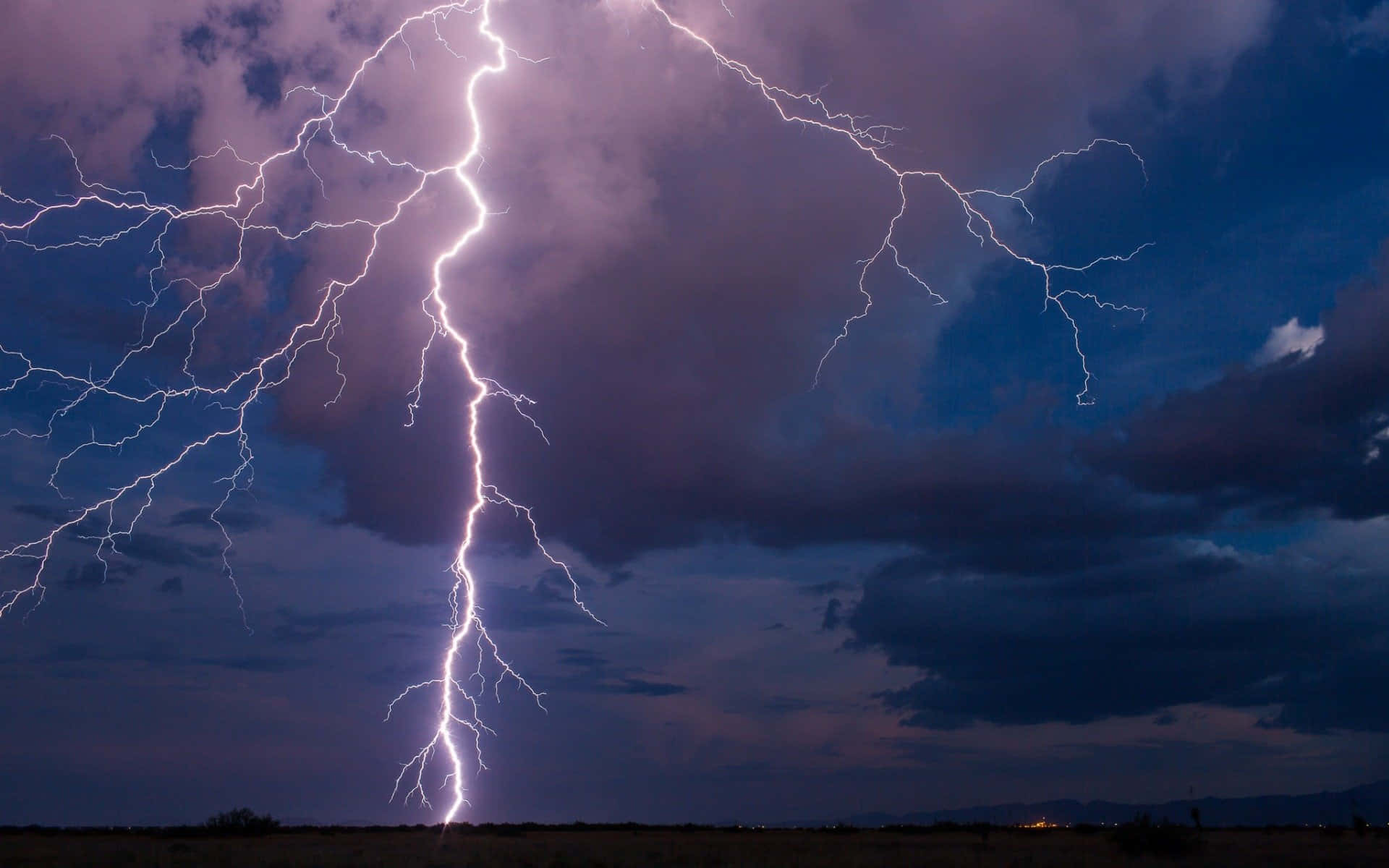In this captivating nighttime photo, the sky is a dramatic tapestry of dark blue and purple clouds. Dominating the scene is a striking lightning bolt, descending from the upper left third of the image and branching into several luminous tendrils, each reflecting hints of purple from the stormy sky. The powerful lightning strike illuminates the otherwise dark landscape below, which appears to be a flat, open expanse resembling a plain or field. The ground itself fades into a nearly indistinguishable blackness, further emphasizing the vivid brilliance of the lightning. Off in the distant background, a solitary building emits a faint electric light, possibly from an office or similar structure, adding a subtle yet intriguing element to the composition. The overall intensity and detail captured in the photo evoke a sense of awe, making it a truly extraordinary shot of nature's raw power.